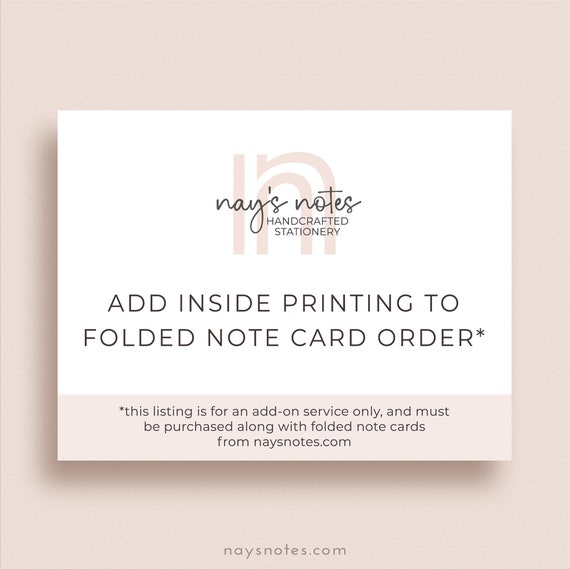This advertisement for Nae's Notes features a primarily white background with a prominent pink logo at the top, highlighting the brand's name, "Nae's Notes," in eye-catching script. Beneath the name, the tagline "Handcrafted Stationery" is displayed in a distinct, elegant font. The main message, "Add Inside Printing to Folded Note Card Order," is emphasized in a larger font, drawing attention to the add-on service. Towards the bottom, the text specifies that this offer is for an additional service only, to be purchased along with folded note cards from the website, NaesNotes.com, which is clearly listed again at the bottom for easy reference. A pink section highlights the asterisk note, ensuring it stands out against the white background. The overall elegant design utilizes shades of pink and light brown to keep a cohesive, visually appealing color scheme.